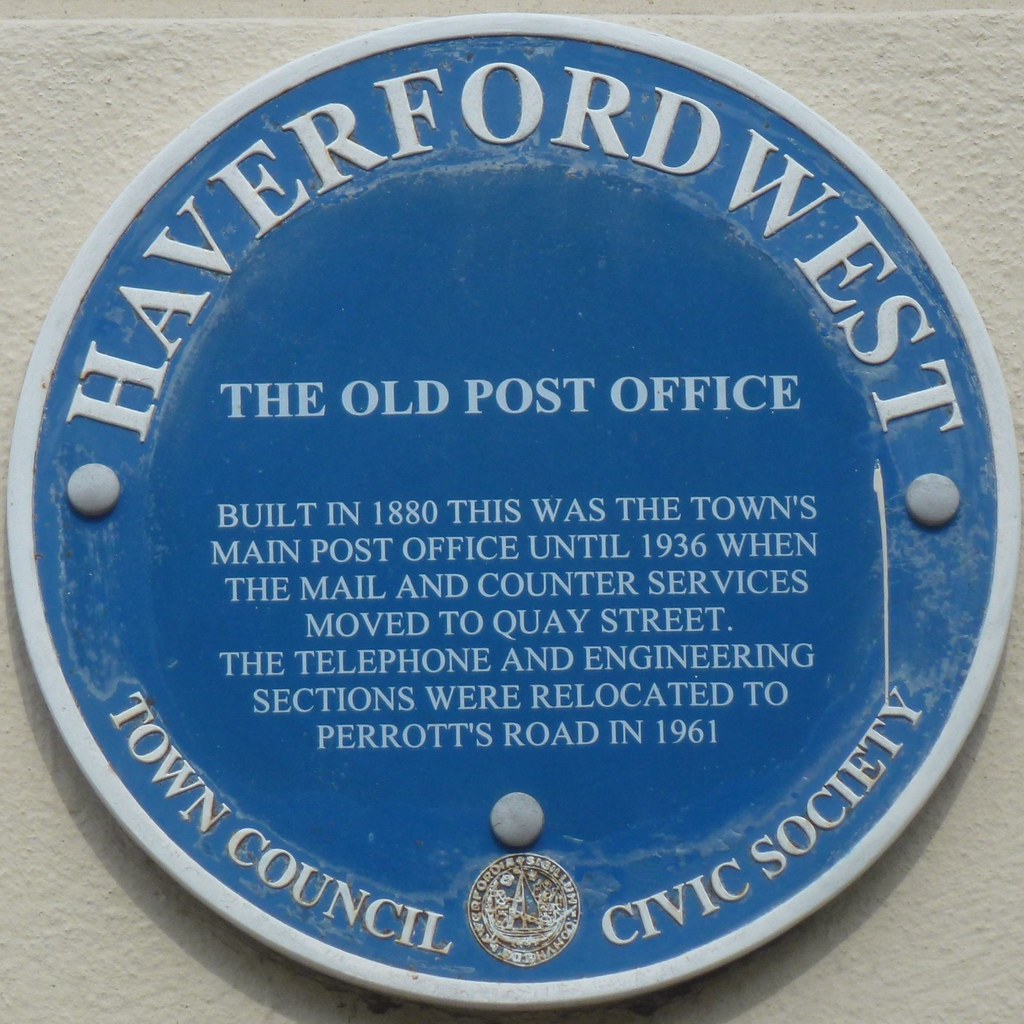The image features a blue circular sign mounted on a beige or white-cream wall. The sign is bordered by a light gray or white edge. At the top, in arched white letters, it reads "Haverford West." Centrally, the sign states "The Old Post Office," followed by a detailed paragraph: "Built in 1880, this was the town's main post office until 1936 when the mail and counter services moved to Quay Street. The telephone and engineering sections were relocated to Parrots Road in 1961." At the bottom, also in arched white letters, it says "Town Council Civic Society," encompassing an ornate silver-colored seal. The sign serves as a historical marker, outlining the significance of the old post office in Haverford West.